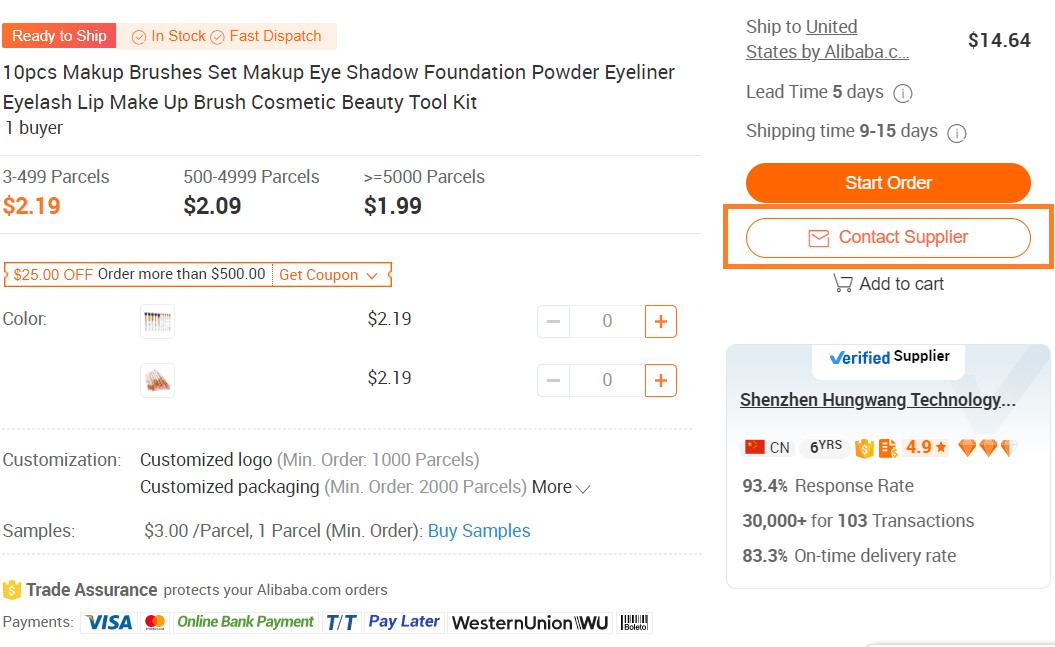Screenshot from Alibaba Purchasing Website

This screenshot captures a purchase page from the Alibaba website, specifically displaying a product listing for a 10-piece makeup brush set. At the top right corner, it notes that the product will be shipped to the United States by Alibaba, though the company's logo is not present. 

The product is described as a "Ready to Ship" item, meaning it is in stock and available for fast dispatch. The detailed product name reads: "10-piece makeup brushes set - makeup, eyeshadow, foundation, powder, eyeliner, eyelash, lip makeup brush cosmetic beauty toolkit."

Pricing details below the product name indicate tiered pricing based on the quantity ordered:
- 1 buyer: Not specified
- 3 to 4,999 units: $2.19 each
- 5,000 units and above: $1.99 each 

Additionally, a special offer is highlighted: "$25 off orders more than 500," with an option to "Get Coupon".

Two color variants of the makeup brush set are shown, though no color has been selected yet, and both are listed at the same price. 

On the right side of the screenshot, there is an orange box highlighting a "Contact Supplier" button, providing potential buyers with the option to reach out directly for more information or negotiation.